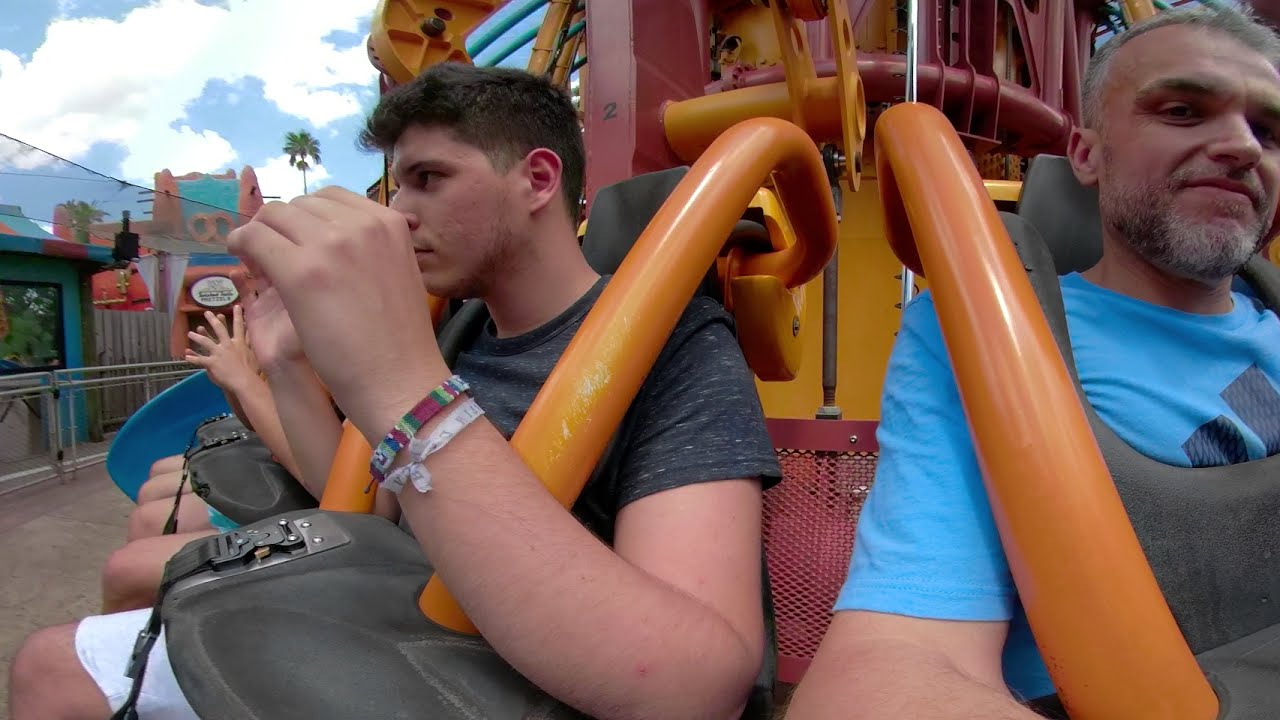The photograph captures an outdoor amusement park ride with several people secured in their seats, ready for the ride to begin. The scene shows a mixture of detailed safety features and the vibrant environment of the park. There are two main individuals in clear focus. The man on the left appears to be in his 20s with short brown hair, wearing a black t-shirt. He is slightly facing left, his arms raised in a bracing posture. The man on the right looks older, possibly in his late 30s or early 40s, with gray hair visible on his head and in his mustache and beard. He is wearing a light blue shirt and looking directly at the camera. Both are secured by thick orange shoulder restraints and a substantial black lap bar. The backdrop includes a circular red and orange ride mechanism, suggesting they are seated on the ride, ready for it to start. The ground below is paved, with a protective guardrail and nearby amusement park structures. The sky above is clear with patches of white clouds, adding to the lively and anticipatory atmosphere.